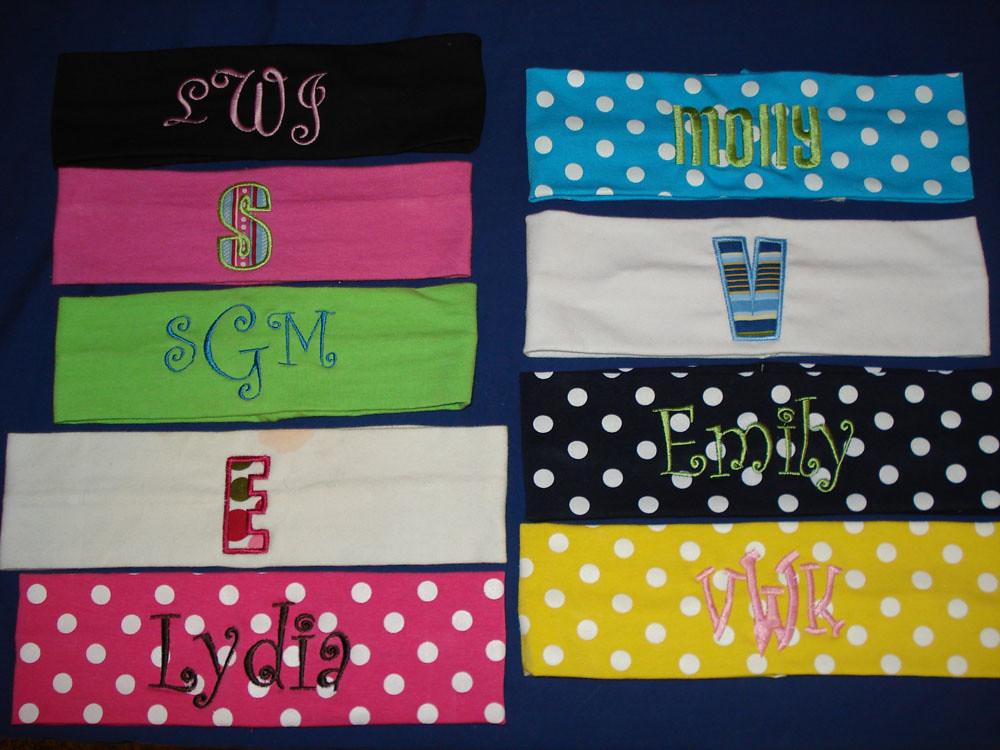The image showcases a collection of personalized, stretchy fabric headbands arranged meticulously against a navy blue background, likely intended for online sale to display the product range. 

On the left side, there are five headbands: The first is black with ornate, swirling pink initials "LWJ". Beneath that is a blue headband, followed by a pink one featuring a multicolored applique of the letter "S." Next is a lime green headband with blue initials "SGM" embroidered in elegant, swirling letters. The final headband in this line is white with a multicolored appliqued letter "E."

On the right side, there are four headbands: The top one is blue with white polka dots, embroidered with the name "Molly" in green. Below it is a solid white headband with a multicolored "V" applique. Next in line is a black and white polka dot headband with the name "Emily" embroidered in green. Finally, the bottom headband is yellow with white polka dots and embroidered with the initials "VWK." 

This detailed arrangement highlights the craftsmanship and personalization options available, making it a compelling display of the product offerings.